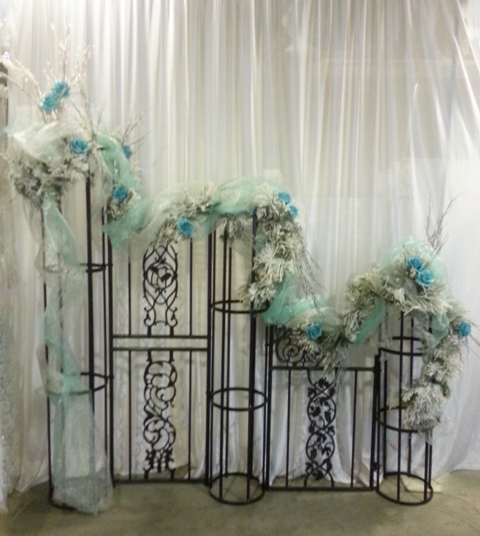The image appears to depict a scene from a wedding celebration. The central focus is on several decorative stands adorned with elaborate arrangements. These stands hold bundles of white flowers interspersed with blue blooms, which seem to be artificial. Surrounding the floral displays are accents of ribbon and cloth, also predominantly white, contributing to the festive and elegant atmosphere. In the background, a pure white curtain further emphasizes the theme of the event, creating a refined and serene backdrop typical of wedding decor. The entire arrangement exudes an aura of joyful celebration and meticulous planning, characteristic of wedding decorations.